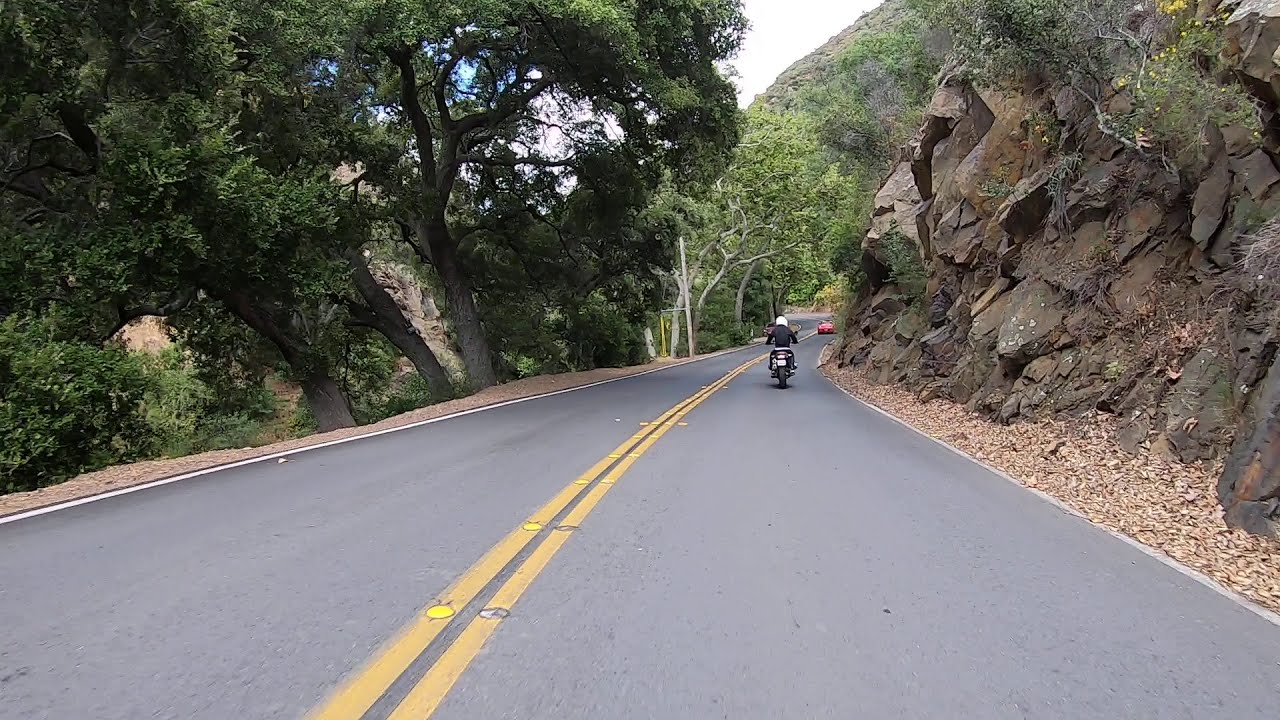The image captures a long, light gray asphalt road that stretches into the distance, bordered by double yellow lines running down its center. Dominating the left side of the road are lush, tall green trees with dense leaves, offering a vibrant contrast to the more barren landscape around them. On the right side of the road, a rugged and jagged rocky mountain rises, its face composed of large, irregular rocks. Some dead leaves and sparse vegetation can be seen at the base of the rock formation. A motorcyclist, dressed in a black jacket and wearing a white helmet, rides along the road. Further ahead, a red car is visible traveling the same direction. The scene is set against a daytime sky, possibly blue with scattered white clouds, adding a serene backdrop to the dynamic elements of the picture.